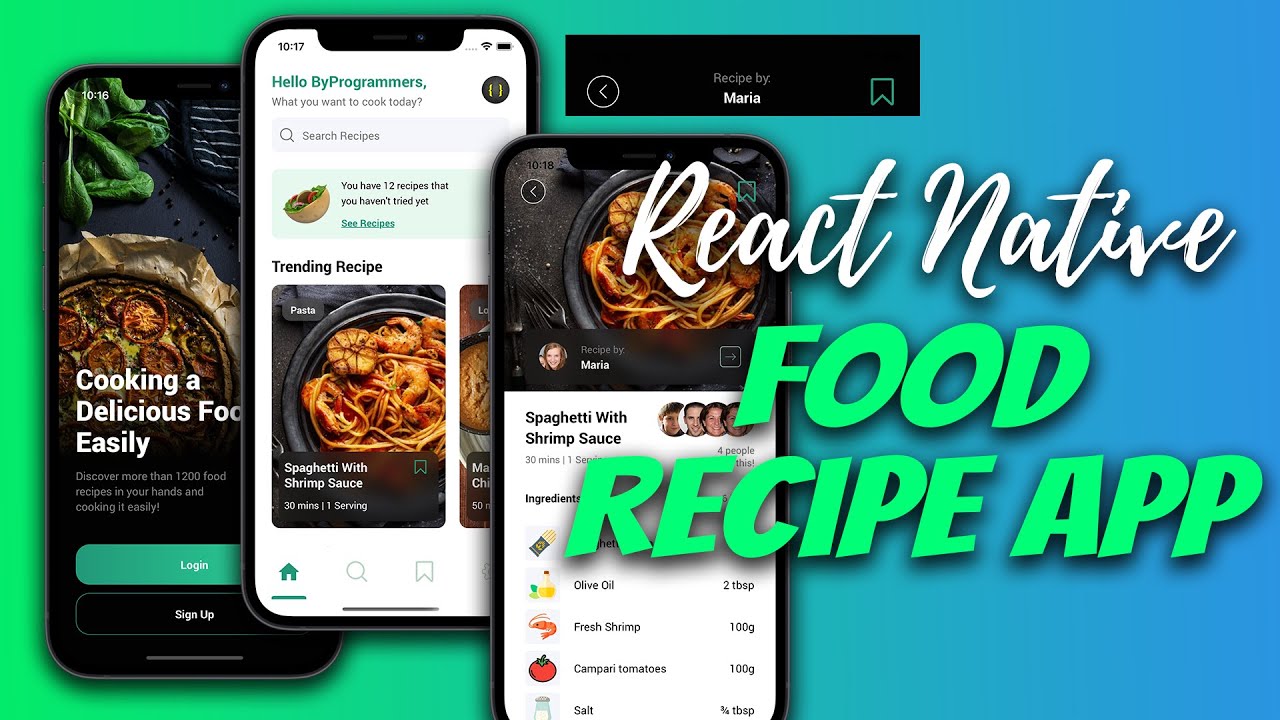The image, designed as a thumbnail for a YouTube video, showcases three vibrant screenshots of a culinary app designed with React Native, perfect for cooking enthusiasts. In a landscape orientation, the app's interface is depicted on three smartphones aligned side-by-side: 

- The left phone displays the login screen with a welcoming caption, "cooking a delicious food easily," superimposed over an image of a bowl of food.
- The central phone stands slightly elevated, revealing the home screen featuring two appetizing bowls of food, with headings “hello by programmers” and “trending recipe” at the top.
- The right phone presents a detailed recipe with ingredients and quantities for “spaghetti with shrimp sauce,” showcasing a top-down view of the dish.

Each screen integrates seamlessly into a gradient background transitioning from green to blue, offering a visually appealing and cohesive design. Positioned at the top of the image, white text reads "React Native" followed by "food recipe app" in bright green. A black rectangle at the top center bears the inscription "recipe by Maria," tying the presentation together with professional clarity and inviting viewers to explore the app’s flavorful possibilities.